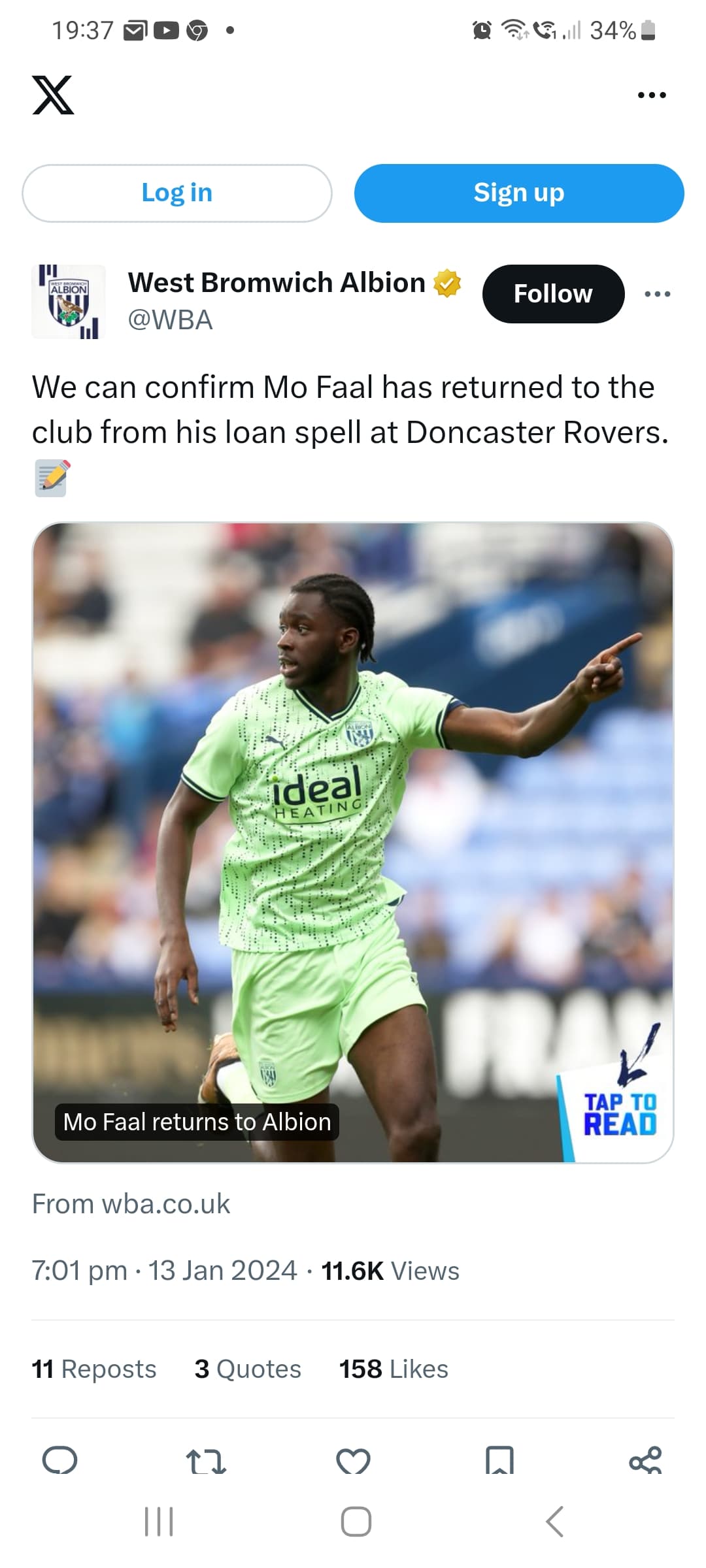Here is a detailed and cleaned-up descriptive caption for the provided image:

---

**Screenshot of a Mobile Application Interface**

The image captures a screenshot of a mobile application with a clean, white background. At the very top, the familiar mobile status icons are visible on the top bar. 

Directly below these icons, on the top left, is a distinctive black logo resembling the letter 'X'. This 'X' features a unique design with a white bar dissecting the line stretching from the top left to the bottom right. 

On the top right corner, three black, horizontally-aligned dots indicate additional options. Below this section, two prominent buttons are displayed side-by-side. The left button is white and pill-shaped, encased in a thin gray outline, with the blue text "Log In" centered within it. On the right, a bright blue pill-shaped button features the white text "Sign Up".

Further down, on the left side, there is a square profile picture with a light gray background. This image includes a black and white shield icon displaying a profile of a person. At the top of the shield, in all caps, the word "ALBION" is inscribed in black text.

To the right of this profile image, bold black text reads "West Bromwich Albion". Beneath this, aligned to the left, is smaller light gray text with the handle "@WBA". Next to this handle, a sun emoji with a white check mark indicates verification.

Adjacent to the handle is a black pill-shaped button with the white word "Follow". Next to this button, three dark gray dots are horizontally positioned, providing more options.

Below this section, stretching across the width of the page, light gray text announces: "We can confirm Mo Faal has returned to the club from his loan spell at Doncaster Rovers." Further down on the left, there is an emoji depicting a gray piece of paper with dark gray lines and a yellow pencil angled across it.

At the bottom of the screenshot, a picture of a soccer player is prominently displayed, completing the visual information on this screen.

---